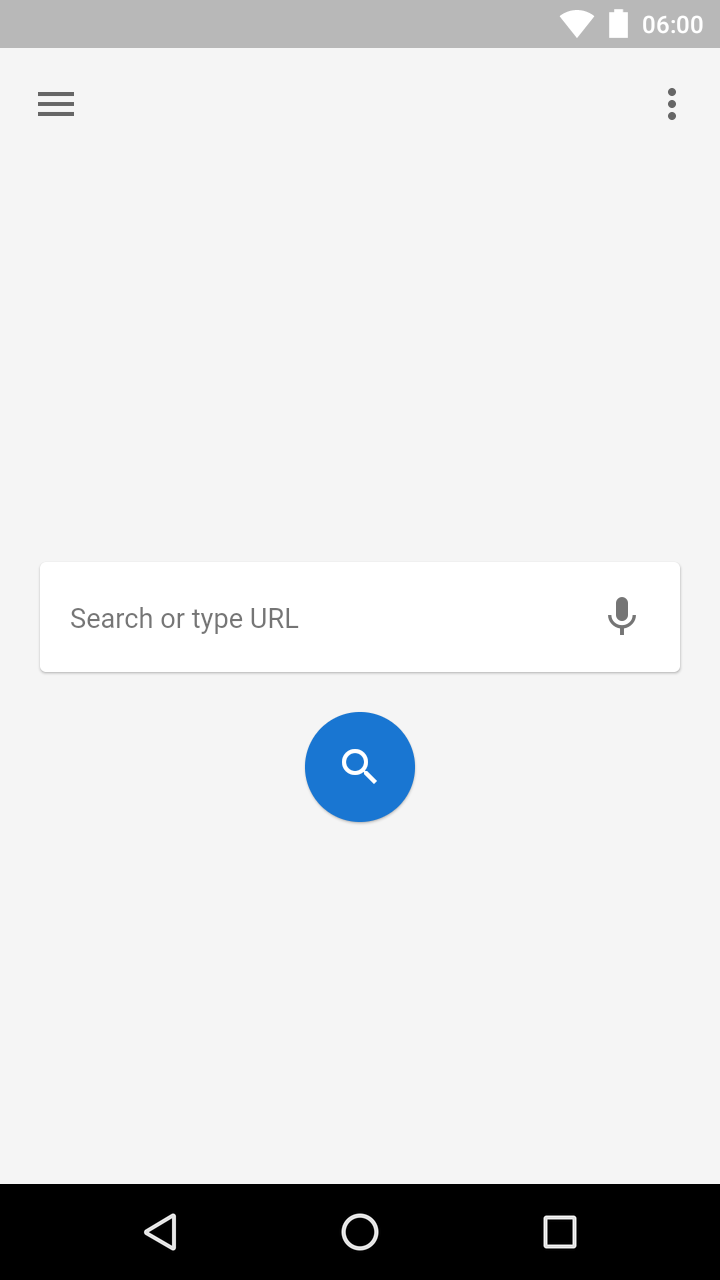The image is a screenshot of a smartphone display. At the top of the screen, occupying the upper one or two centimeters, there is a gray status bar. On the right end of this status bar, white icons indicate the phone's Wi-Fi connection, battery level (displayed vertically), and the time, which is 0600 hours. 

Below the status bar, the screen has a beige background. On the top left corner, there is a menu icon represented by three horizontal lines. Opposite to this, on the right, are three vertically-aligned dots, also known as the kebab menu icon.

Central to this display is a search bar where users can type a query. It reads "Search or type URL" with a small microphone icon adjacent to it, suggesting the option for voice search. Below this bar, there's a blue circle featuring a magnifying glass, symbolizing the search button.

At the very bottom of the screen, there's a black navigation bar about two or three centimeters in height. This bar contains three evenly spaced icons: a triangle on the left, a circle in the center, and a square on the right. These icons are white outlines, not filled in, allowing the black background to be visible through them.